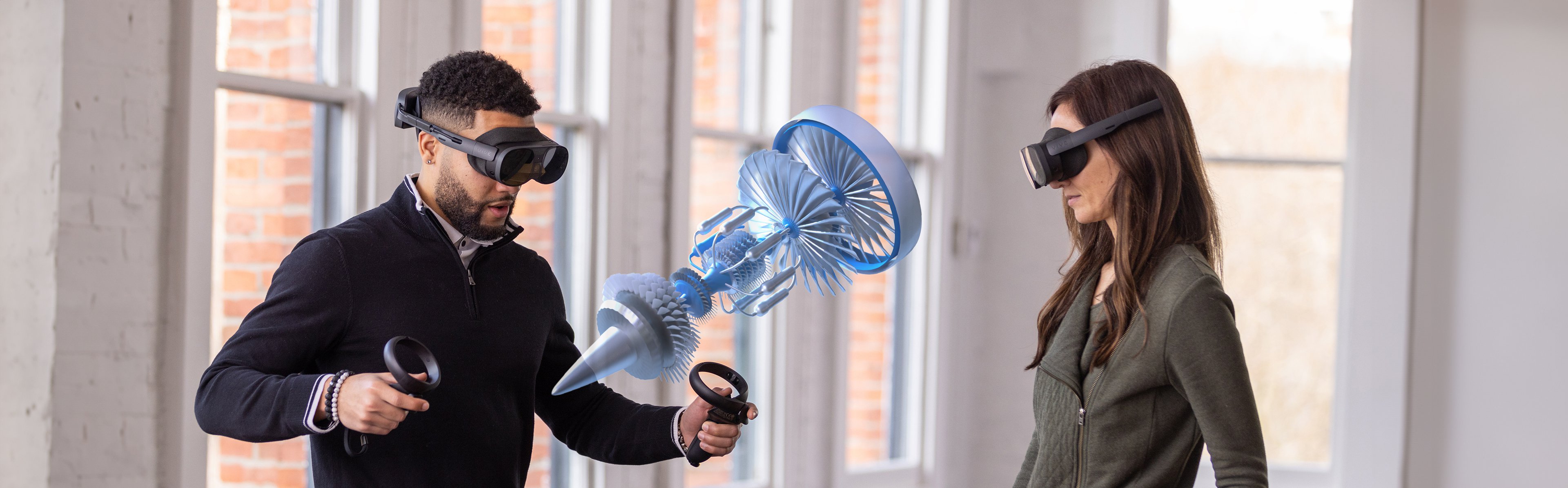The photograph, in a wide rectangular format, captures two individuals immersed in a virtual reality experience. On the left, a black man with short hair and a black beard wears a black zip-up sweater and holds VR controllers with circular rings in his hands. Beside him on the right, a white woman with brunette hair dons a dark gray long-sleeved shirt. Both participants are equipped with black VR headsets, engrossed in observing a 3D model of a jet engine that appears virtually between them. The setting is an indoor space with large windows, through which a brick exterior can be seen, suggesting a cozy living room or common area within an apartment building.